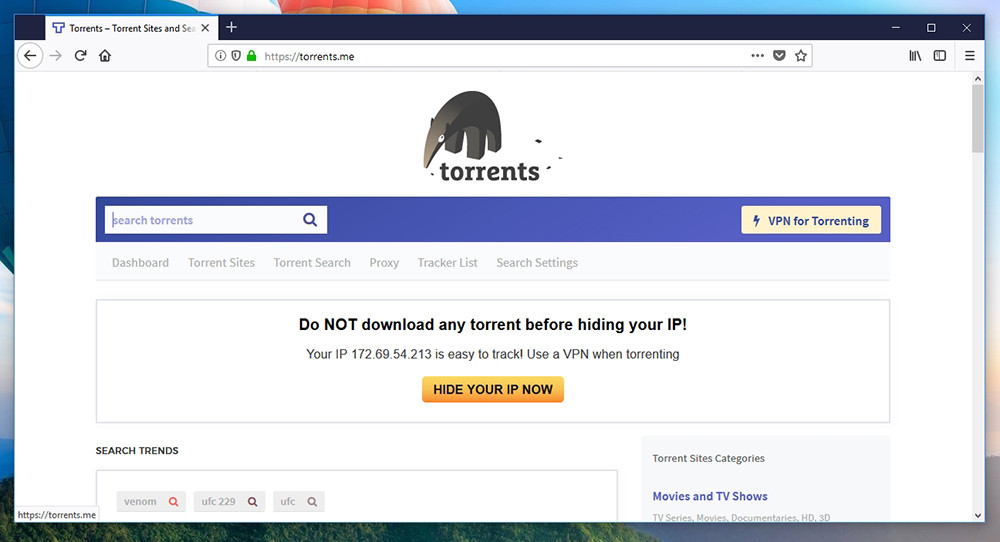The image shows a screenshot of a computer screen displaying a website on a browser. Surrounding the screen are thin borders of the computer’s background, which features a hot air balloon against blue skies with hints of orange. The browser tab reads "torrents - torrent sites and something else." Below the address bar, identifiable icons include left and right arrows, a refresh arrow, and a house icon.

The website in the screenshot is torrents.me. Prominently at the top is a grayscale cartoon image resembling an aardvark or anteater, followed by the word "torrents" in dark gray letters. Below this, a blue rectangular section spans across the screen, with a search bar on the left side labeled "search torrents" and a text on the right side stating "VPN for torrenting." 

Further down, a navigation bar lists various categories: Dashboard, Torrent Sites, Torrent Search, Proxy, Tracker List, and Search Settings. Below this, a warning message reads: "Do not download any torrents before hiding your IP! Your IP 172.69.54.213 is easy to track. Use a VPN when torrenting." A notable yellow rectangular button beneath the warning says "Hide your IP now," inviting users to take protective action.